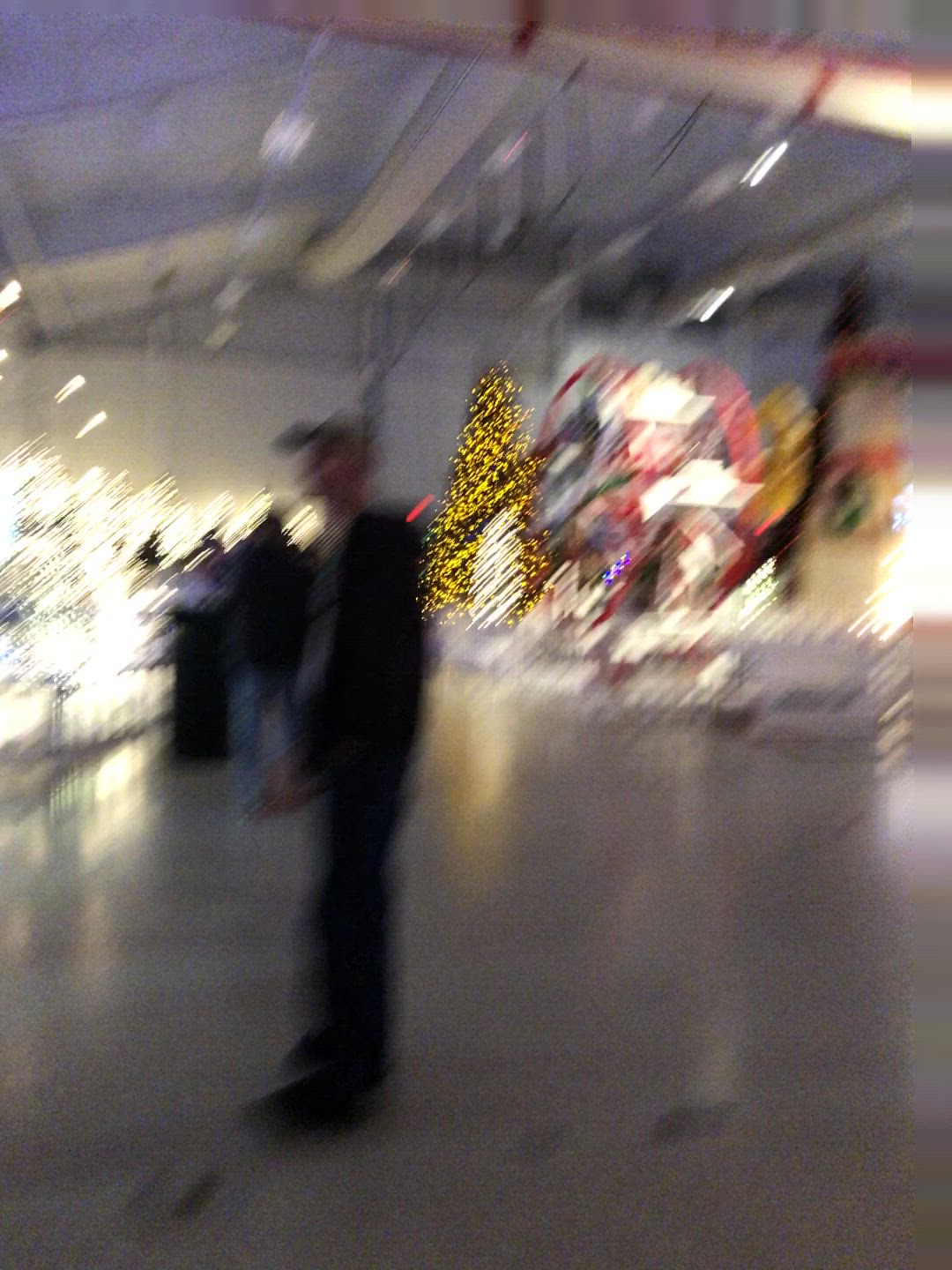This photograph, despite its blur, captures a vibrant Christmas-themed event inside a large, industrial warehouse. The dimly lit setting typifies an indoor festive attraction, likely designed for children, featuring numerous Christmas decorations. Dominating the scene are multiple Christmas trees adorned with golden lights and possibly inflatable snowmen. Overhead, the warehouse's structure is visible with steel beams, fluorescent lights, ductwork, and piping adding to the industrial aesthetic. In the foreground, slightly off-center to the right, stands a person in black attire, including a hat and jeans, surrounded by several others in the background, all somewhat obscure due to the photo’s blurriness. Also notable are strings of Christmas lights scattered throughout, and what appears to be the outline of a Ferris wheel-like structure on the left side. The concrete floor and the general festive arrangements contribute to the feel of a Christmas bazaar or celebration, likely filled with attractions designed to delight visitors during the holiday season.